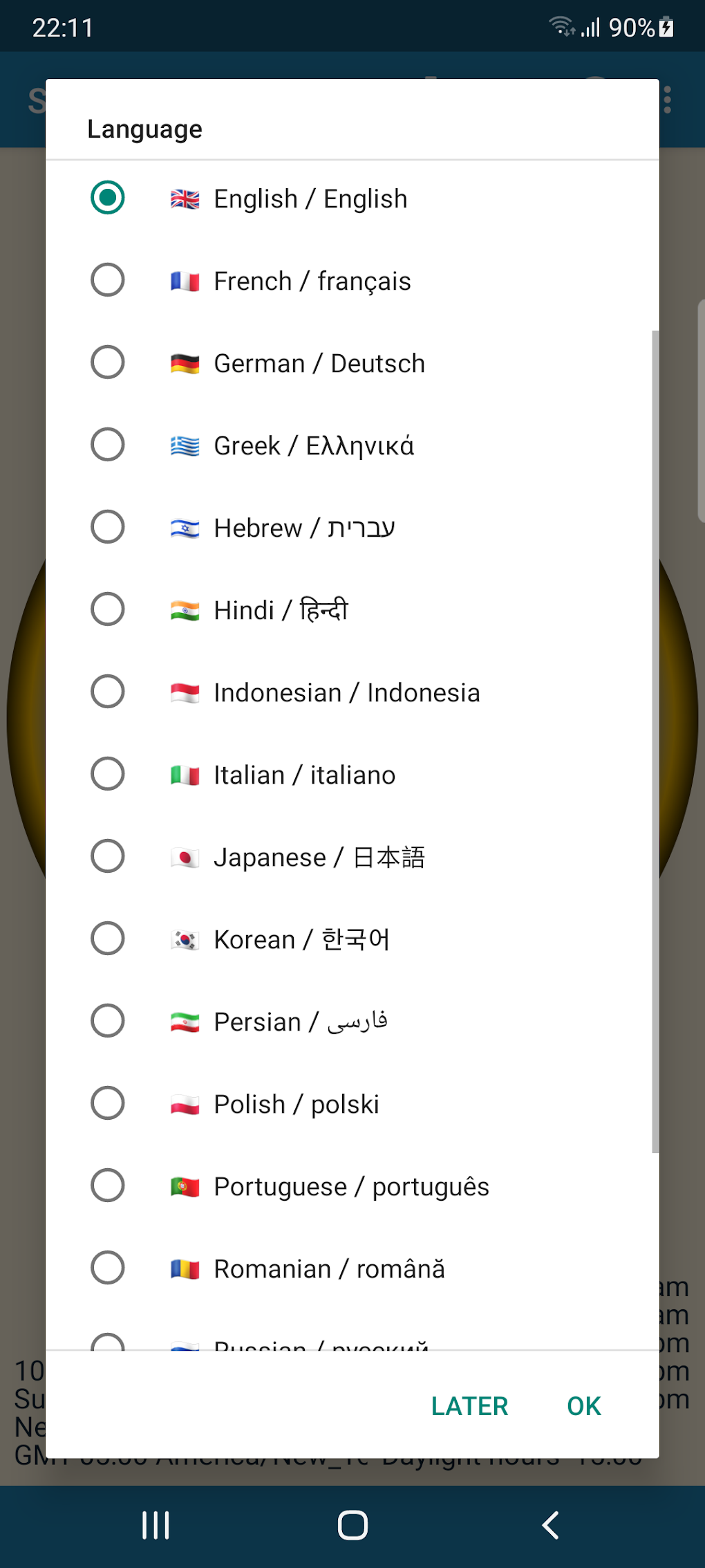A person is using a smartphone, specifically engaging with what appears to be a translation application. The interface prominently features a pop-up dialog box prompting the user to select a language. Currently, "English" is selected, associated with the flag of the United Kingdom. The pop-up offers a wide range of languages to choose from, including French, German, Greek, Hebrew, Hindi, and many others, displayed alongside their respective national flags.

The pop-up nearly obscures the entire screen, making it difficult to discern the background image, which seems to depict a large yellow sphere. The device shows a battery level of 90%, full cellular signal bars, but a weak Wi-Fi connection. At the bottom of the pop-up, there are two buttons: "OK" and "Later", inviting the user either to confirm their selection or to delay the choice.